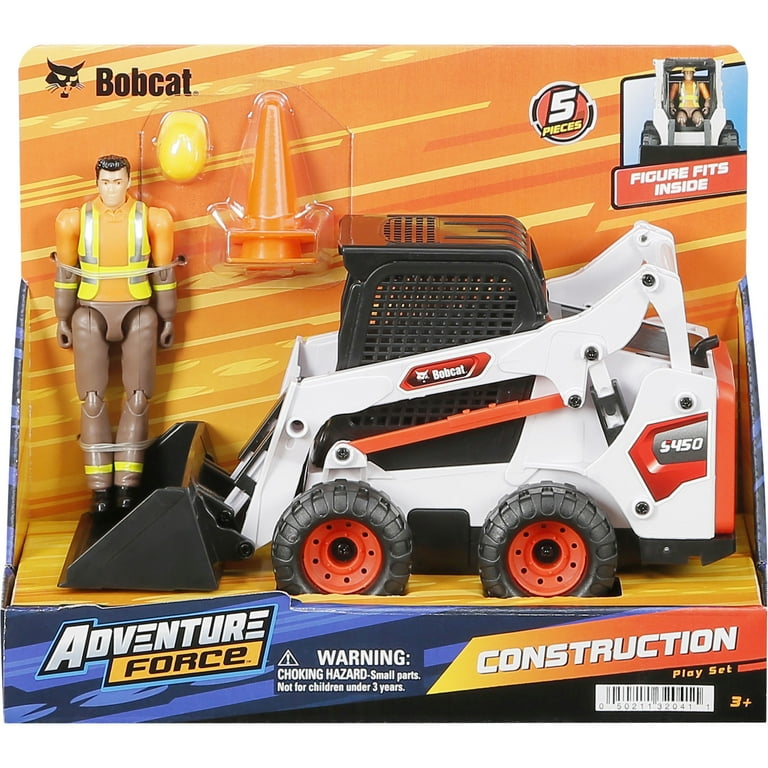This detailed image showcases a children's toy construction playset, prominently featuring a white Bobcat construction vehicle with black wheels, a black shovel, and a black passenger area, adorned with red trim. The packaging highlights the Bobcat brand with a logo featuring a black bobcat face and text in the top left corner. The vehicle is part of an Adventure Force playset, as indicated in the bottom left corner of the box, which also includes a warning about small parts posing a choking hazard for children under three years.

The toy set is displayed in a cardboard box, with the inside of the box having an orange background and the exterior base being blue. The package also includes a construction worker figure with articulated limbs, featuring a yellow vest, orange shirt, brown pants with yellow stripes, black boots, and a yellow hard hat. The figure is zip-tied to the packaging and is shown to fit inside the vehicle, as demonstrated by an image on the top of the box.

Accompanying the set are two orange traffic pylons to enhance the construction play experience, summing up to the five advertised pieces. The bottom right corner of the box states "construction playset" and includes a white barcode, while safety warnings and age recommendations (for children three years and older) are clearly marked. The overall background design of the packaging incorporates an orange and yellow street-themed pattern with stripes.